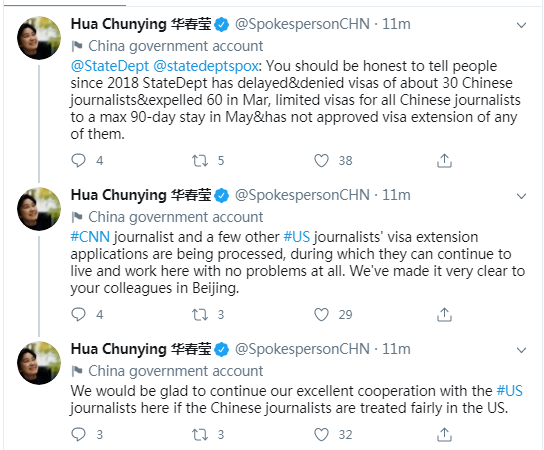Captured from a cell phone screen, this image showcases a conversation involving a verified Chinese government account. The account holder's name is spelled "Haihua Chunying" (H-A-I-H-U-A C-H-U-N-Y-I-N-G), followed by a beautiful Asian script, and is marked with a verification badge. Their handle, "@SpokespersonCHN," indicates that they are an official State Department spokesperson for China. The account’s profile picture shows an individual with dark hair looking upwards and smiling, though their gender is not immediately clear.

The post is timestamped "11 minutes ago" and includes a formal statement addressing the U.S. State Department's treatment of Chinese journalists. It states that since 2018, the State Department has delayed and denied visas for around 30 Chinese journalists, expelling 60 in March, and limited all Chinese journalists to a maximum 90-day stay since May, with no visa extensions approved. A follow-up comment clarifies that visa extension applications for affected journalists are being processed, during which time they can continue to live and work in the U.S. with no issues, adding that this has been communicated clearly to colleagues in Beijing.